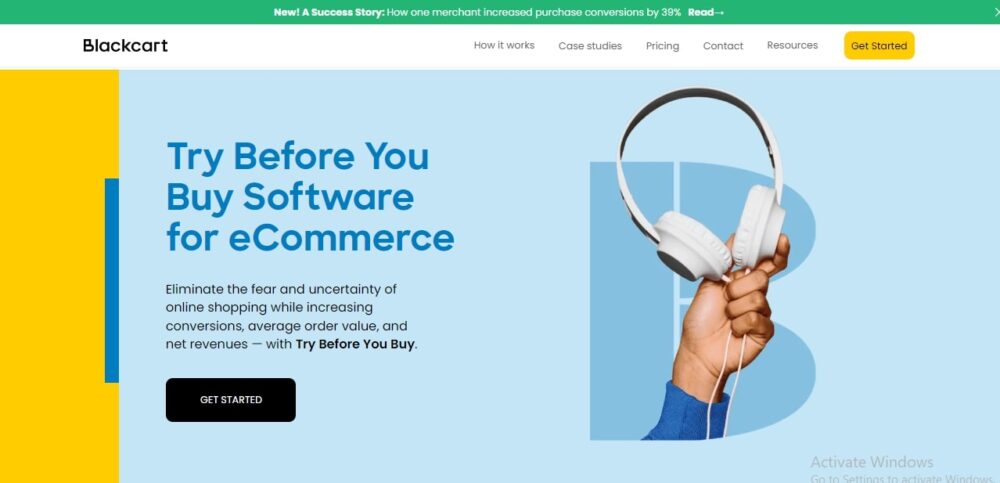The image depicts a sleek, black-themed website for a service related to try-before-you-buy software tailored for e-commerce. 

At the very top, there is a thin green line featuring text in white font that reads, "New Success Story: How one merchant increased purchase conversions by 39%." This section includes a "Read" button accompanied by a forward-pointing arrow icon.

Below this, on the left side, the navigation menu appears within a white bar. The title "Black Card" is displayed in bold black font. The menu options include: "How it Works," "Case Studies," "Pricing," "Contact," and "Resources." There is also a prominent "Get Started" button with a yellow square and yellow background.

The central portion of the website highlights the primary offering—try-before-you-buy software aimed at e-commerce platforms. This section contains a brief description of the software's benefits and another "Get Started" button, inviting users to take action.